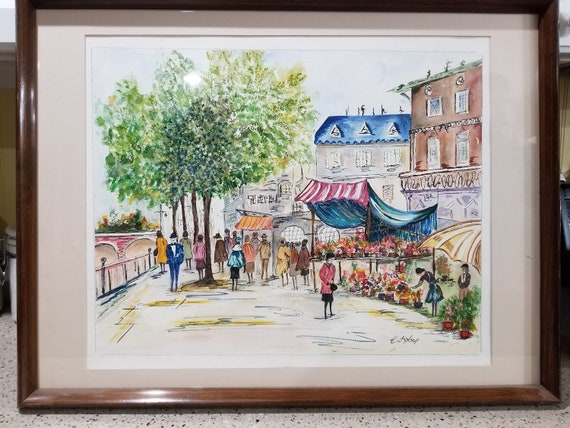A color photograph of a framed Victorian-style illustration depicts a bustling market scene set in a quaint town square. The thin brown wooden frame is complemented by an ivory-colored mat, enhancing the central artwork. The medium, possibly watercolor or colored pencil, captures a vibrant street filled with townsfolk and market stalls. In the background, tall trees and a river with a guardrail contribute to the picturesque setting, complete with a bridge to the left.

The detailed illustration showcases a variety of architectural and human elements. On the right side, two buildings stand prominently: one brown and another with a blue roof. Nestled between these structures is a lively market area adorned with red and blue awnings. Various flower pots and bouquets add splashes of color, attracting the attention of a woman in a red jacket, black skirt, and black hat, who examines the floral displays. Nearby, a shopkeeper tends to the flowers.

In the midst of the scene, numerous pedestrians are depicted strolling about, rendered in different hues like blue, pink, and red, but without distinct facial features. A man in a blue suit and hat strides purposefully towards the viewer, adding a dynamic element to the composition. The illustration beautifully captures a moment in time, blending architectural details, natural elements, and the vibrant life of a market in a charming town.